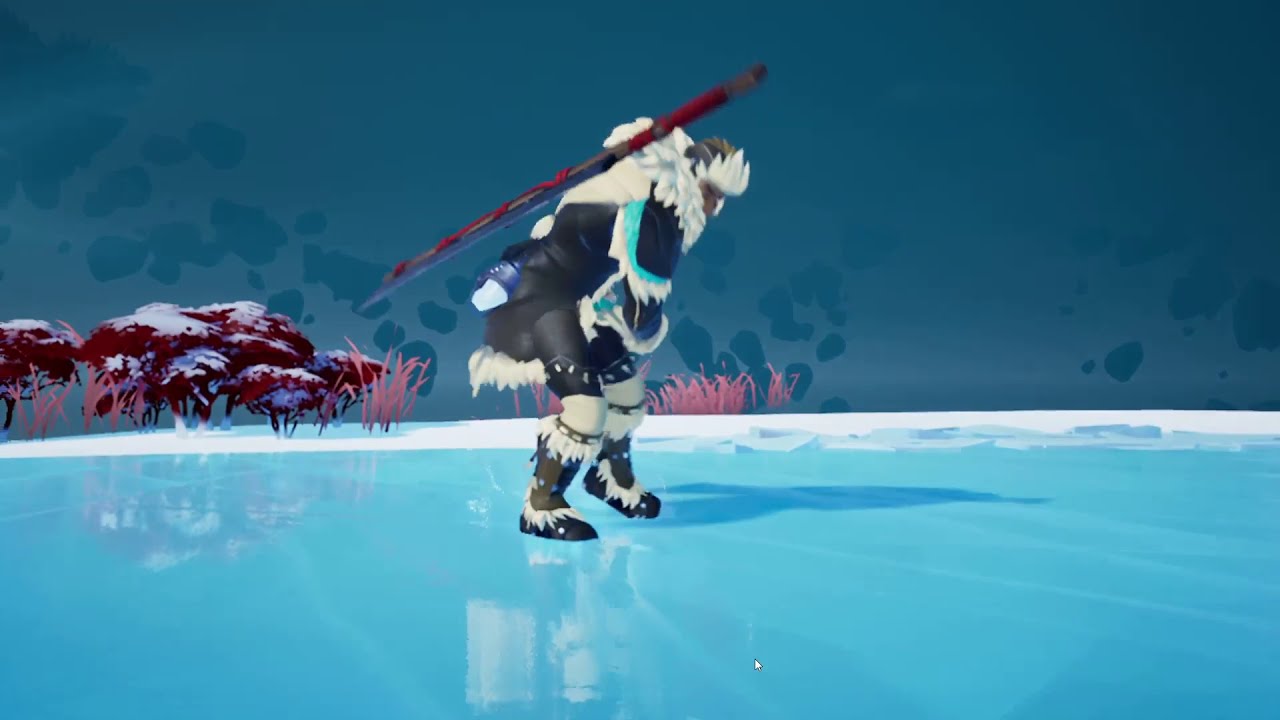An animated 3D figure stands on a light blue, solidly frozen lake, their reflection subtly visible in the ice beneath them. This human-like character is clad in winter gear: a dark jacket with fur accents around the collar and bottom, dark pants, and black boots lined with fur. They wear a white fur-trimmed hat and a white scarf. Strapped to their back is a long, spear-like pole, predominantly red with some gray and brown elements. Surrounding the figure, the ice is framed by snow-covered areas where pinkish, reddish, and purple trees and bushes grow. Snow-capped trees and a foggy white, snow-covered mountain with black rocky outcrops complete the wintry, arctic-like landscape.